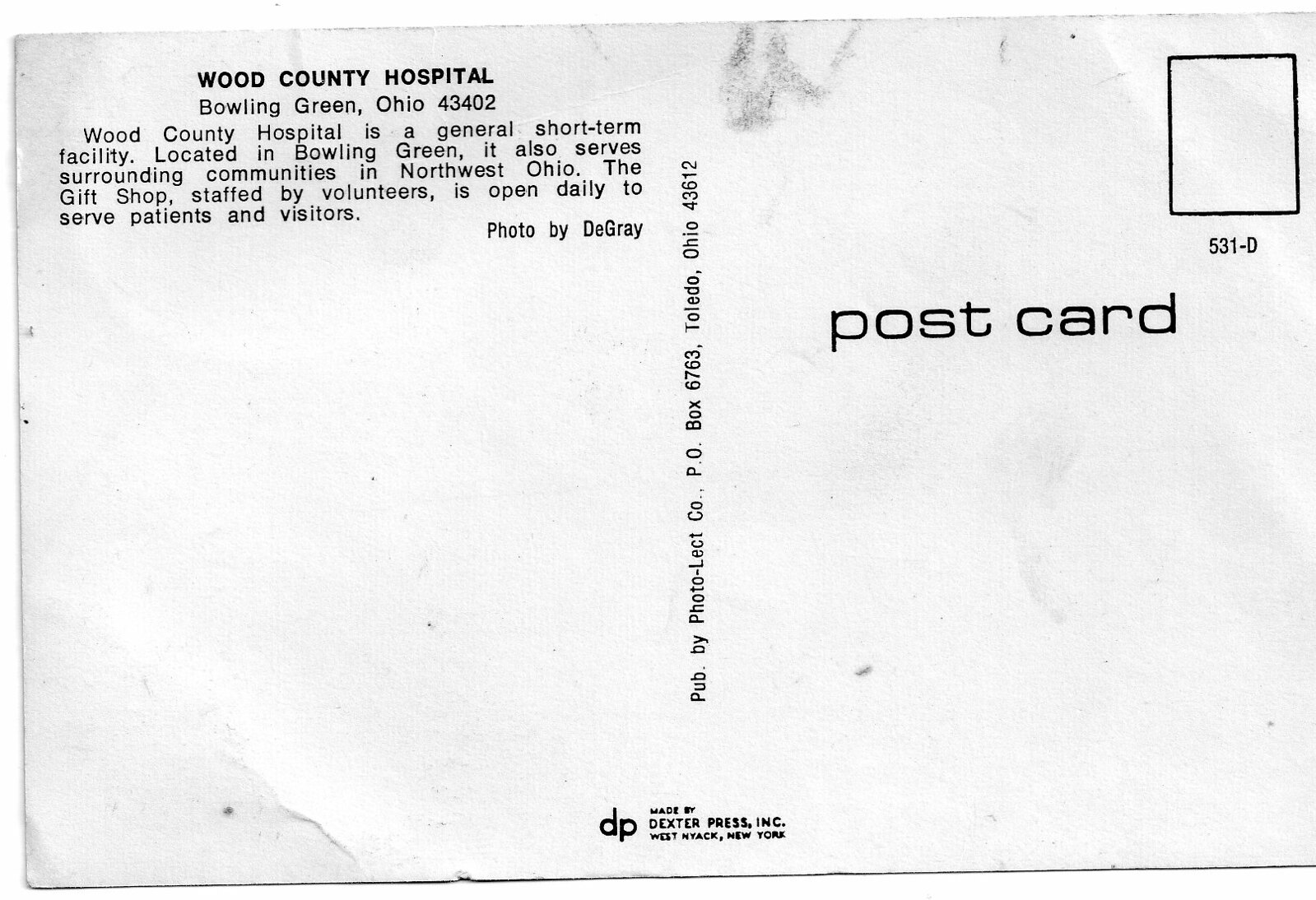This horizontally aligned rectangular postcard, likely from an earlier era, bears visible signs of age with creases and smudges on its surface. The upper portion of the card features a blank black-outlined square in the top right corner labeled "531-D," designated for a stamp. In the upper left corner, bold text declares "Wood County Hospital," with "Bowling Green, Ohio 43402" centered directly beneath it. Below this, the card describes Wood County Hospital as a general short-term facility in Bowling Green that also serves the surrounding communities in Northwest Ohio. It mentions a gift shop, staffed by volunteers, open daily for patients and visitors. The phrase "photo by DeGray" appears underneath this description.

In the middle of the card, vertically aligned text reads "Published by PhotoElect Company, P.O. Box 6763, Toledo, Ohio 43612." The bottom center features the initials "DP" and the makers' mark, "Made by Dexter Press, Inc., West Nyack, New York." The left middle and lower portions of the postcard remain blank, marred only by some wrinkles and smudges, reinforcing its worn, vintage appearance. This back view suggests that any image related to this postcard would be on the unseen front side.